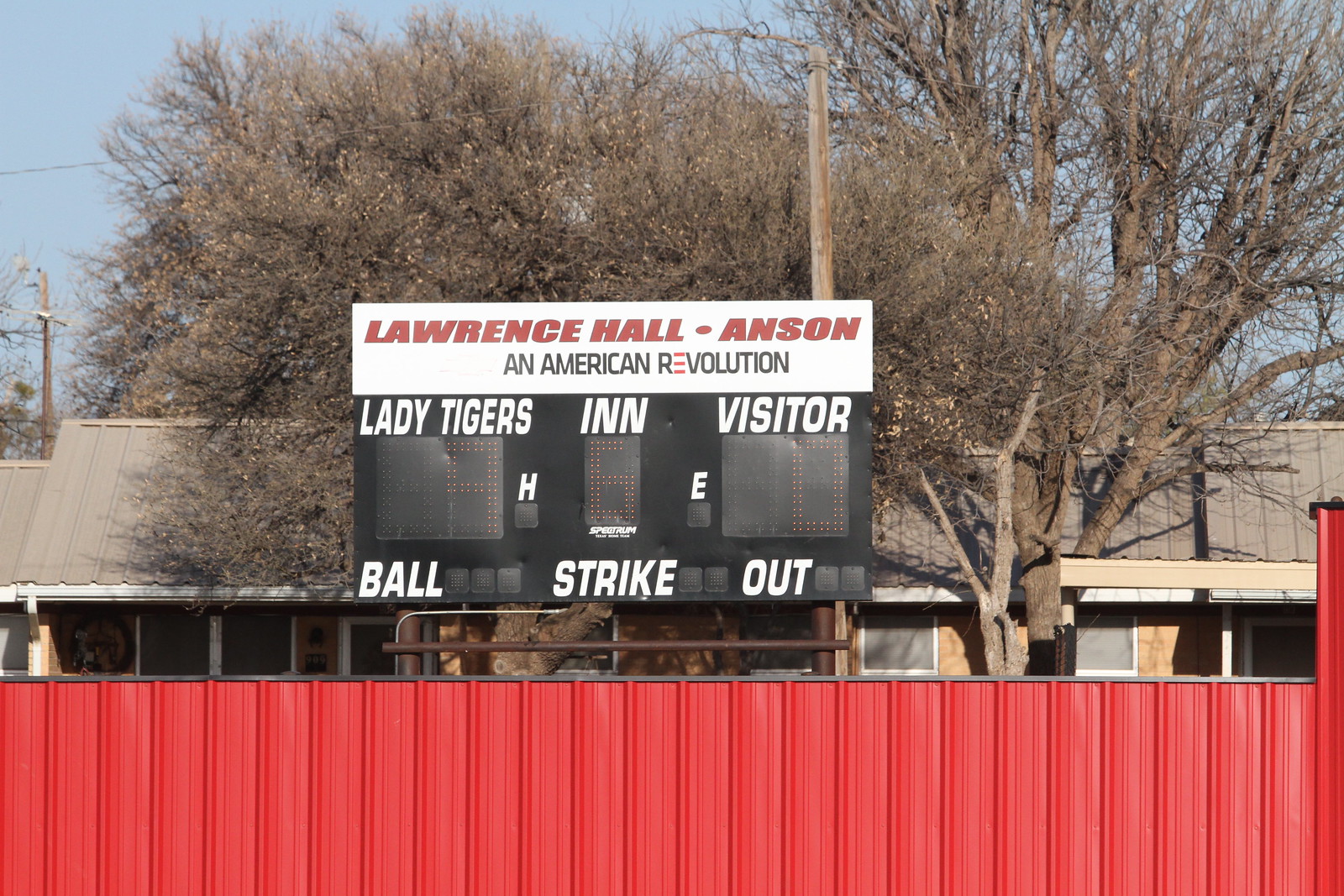This vibrant color photograph captures a bright, sunny day with a deep blue, cloudless sky, hinting at either winter or early spring as the leafless trees line the backdrop. Dominating the center is a black scoreboard, with several details clearly visible despite the intense daylight. 

At the top of the scoreboard, bold red letters display "Lawrence Hall" followed by a circular emblem, and then "Anson." Just beneath, "All-American Revolution" is inscribed in black, with the letter 'E' standing out in red. Below, the scoreboard displays the game's progress: "Lady Tigers" lead with a score of 9, against "Visitor" at 0. It's the 6th inning as indicated by the white letters 'IN' on a black background. The sections for balls, strikes, and outs remain blank.

A striking red wooden fence runs horizontally across the bottom of the image, positioned right in front of the scoreboard. The photograph also features some subtle details including a tan A-frame rooftop and distant telephone lines, adding depth to the scene.